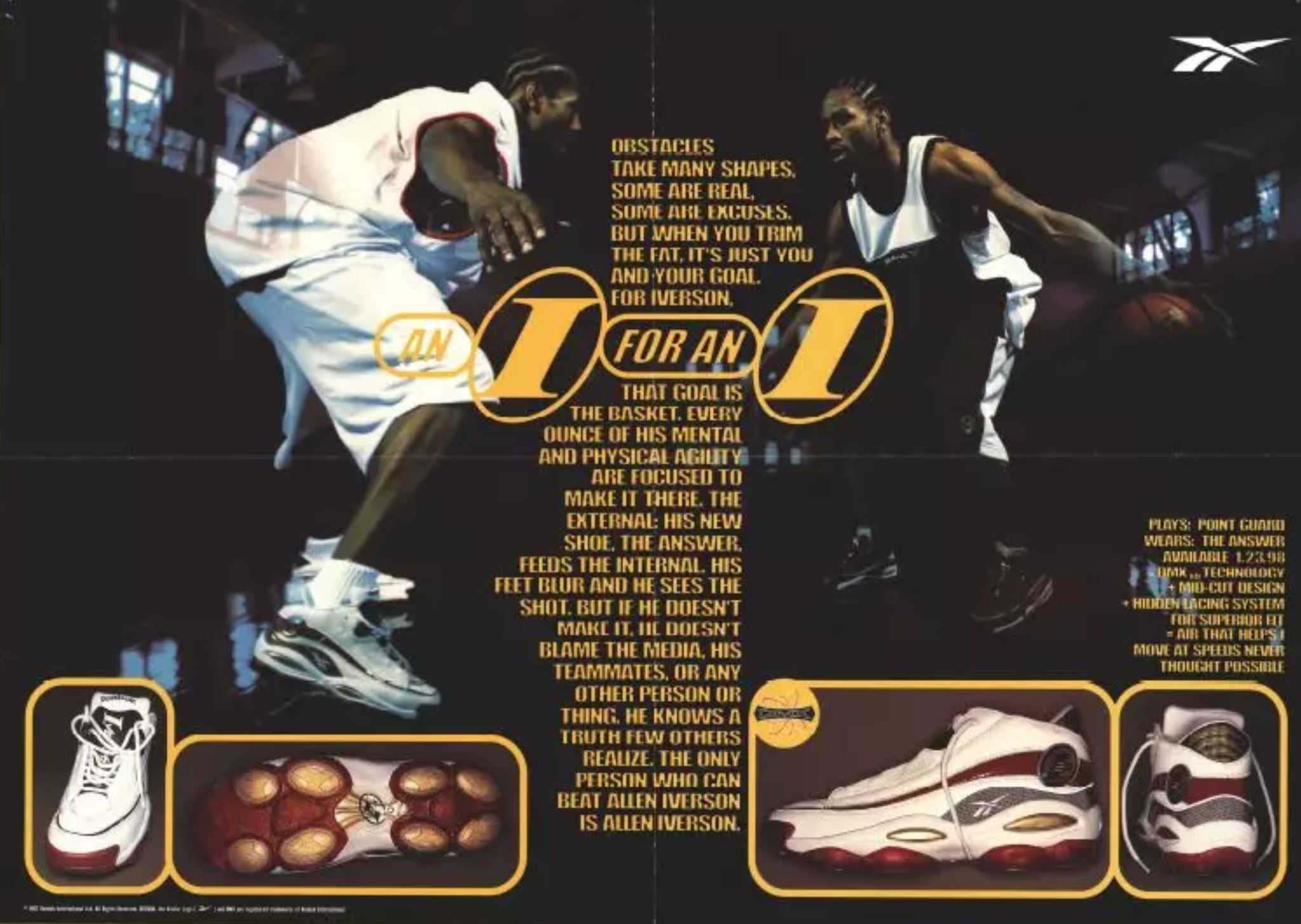The poster is an advertisement for basketball shoes featuring two African-American basketball players, both dressed in white basketball jerseys and shorts, facing off on a dimly lit basketball court. The dark brown background contrasts with bold yellow text at the center that reads: "Obstacles take many shapes. Some are real. Some are excuses. But when you trim the fat, it's just you and your goal." The text continues, emphasizing that for Allen Iverson, the goal is the basket and he channels every ounce of mental and physical agility to make it there. The poster underscores that Iverson's new shoe, "The Answer," enhances his internal drive and focus. It further highlights that Iverson holds himself accountable, knowing that the only person who can defeat him is himself.

At the bottom of the poster, there are detailed images of Iverson's new sneaker from different perspectives: a full-on front view, a sole view, a side view, and a heel view. The sneaker, predominantly white with red, gold, and black accents, features eight gold pads on the sole, which may provide added cushioning. Tie-up laces complete the design, emphasizing its suitability for basketball. Though some additional small text appears in the bottom right corner, it is difficult to read due to its size.